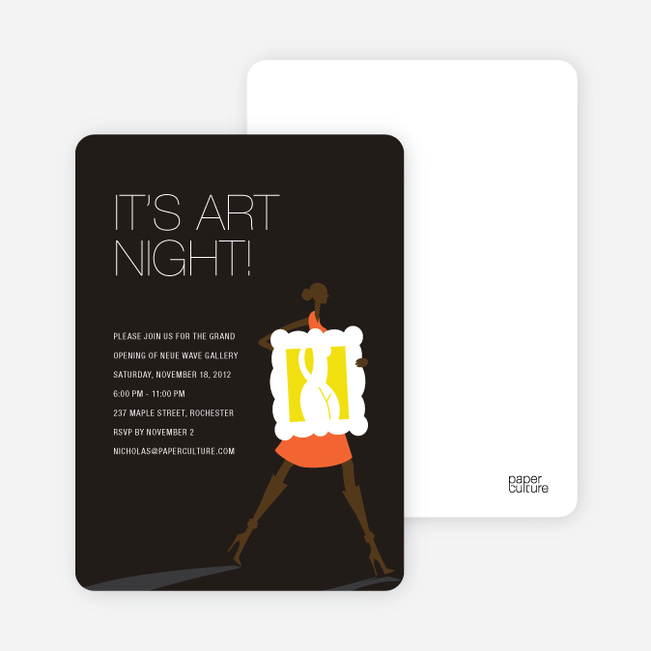The image features three distinct components arranged on a light gray background. The main component is a black poster with a black background that announces an event: "It's Art Night! Please join us for the grand opening of the New Wave Gallery, Saturday, November 18, 2012, 6-11pm, 237 Maple Street, Rochester. RSVP by November 2." Below this text, there is information about NicholasPaperCulture.com. To the right of the text, a stylized cartoon silhouette of a woman with her hair in a bun is depicted holding a framed piece of art showcasing a graphic representation of a naked figure. She is wearing knee-high boots with five-inch heels. Another element of the image is a white paper or page that appears to be underneath the black poster. This white page is mostly blank except for the lower left corner, which simply says "Paper Culture." The overall arrangement is set against a purely light gray background, giving the components a layered appearance.